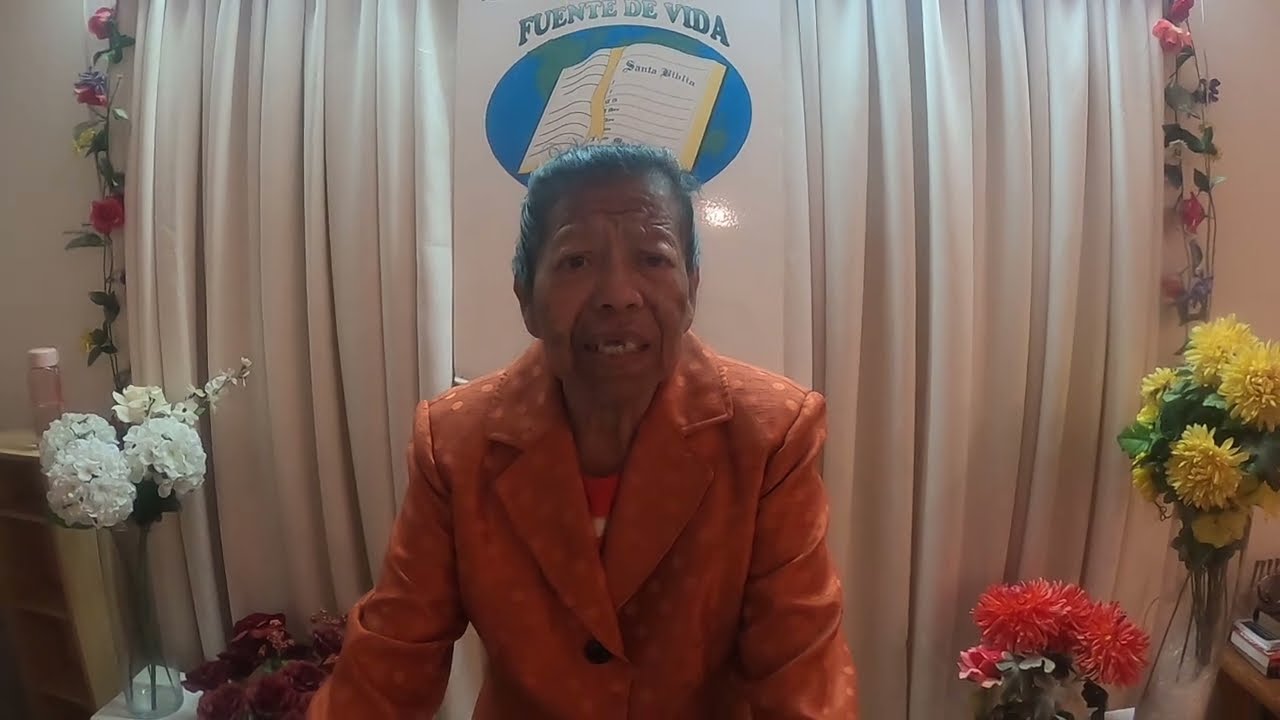An older person with gray hair and darker, mostly wrinkled skin stands in the center of the image, looking straight forward. They are dressed in an orange polka-dotted jacket with slightly lighter orange polka-dots and an orange t-shirt underneath. Behind them, a white curtain serves as a backdrop, adorned with a sign that reads "FUENTE DE VIDA" above a cartoon graphic of a book resting on a green and blue globe. Flanking them are various floral arrangements: to the right, a clear vase holds yellow flowers with green stems, and next to it, a bouquet of orange flowers with green stems. On the left side of the image, white flowers, including hydrangeas and possibly a white rose, are displayed. Additionally, artificial vines with yellow, purple, and pink flowers entwine along the curtain in the background.